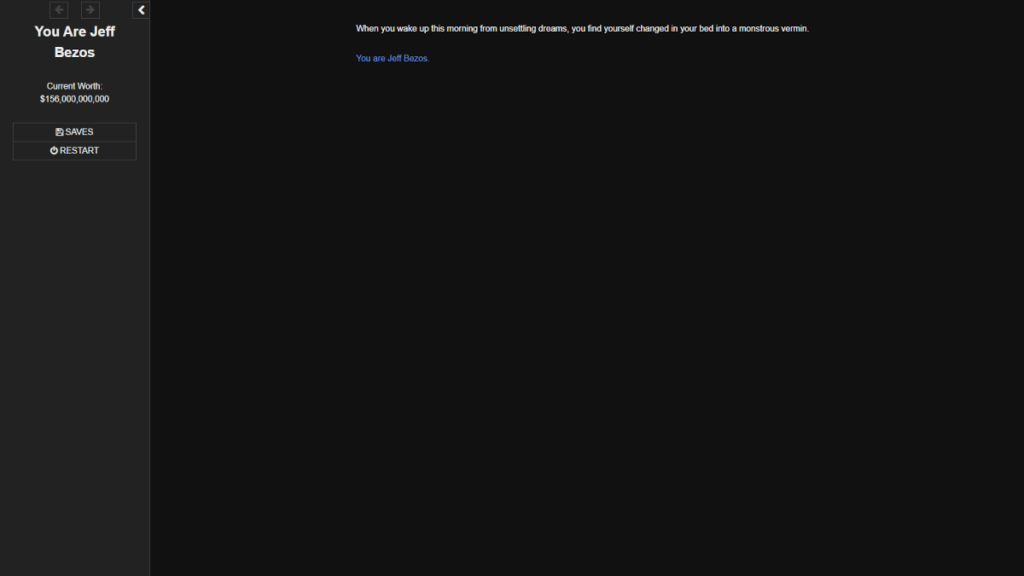The image is a computer screenshot predominantly featuring a black background. On the left side, there is a gray panel. At the top of this panel, a message reads: "For Jeff Bezos, connect with something worth $156 billion." Below this message are two buttons: the top button is labeled "saves," while the bottom one is labeled "restart."

To the right of the gray panel lies a large black area that forms the majority of the image. This black section has a rectangular shape, extending longer horizontally than vertically. At the top center of this black background, there are small, blurry white words that are somewhat difficult to make out, but partially read, "We make you up." Further down, the text becomes clearer, stating, "You find yourself changed in your bed." In a more prominent blue font below this text, the caption reads, "You are Jeff Bezos," with the letters "Y," "J," and "B" capitalized.